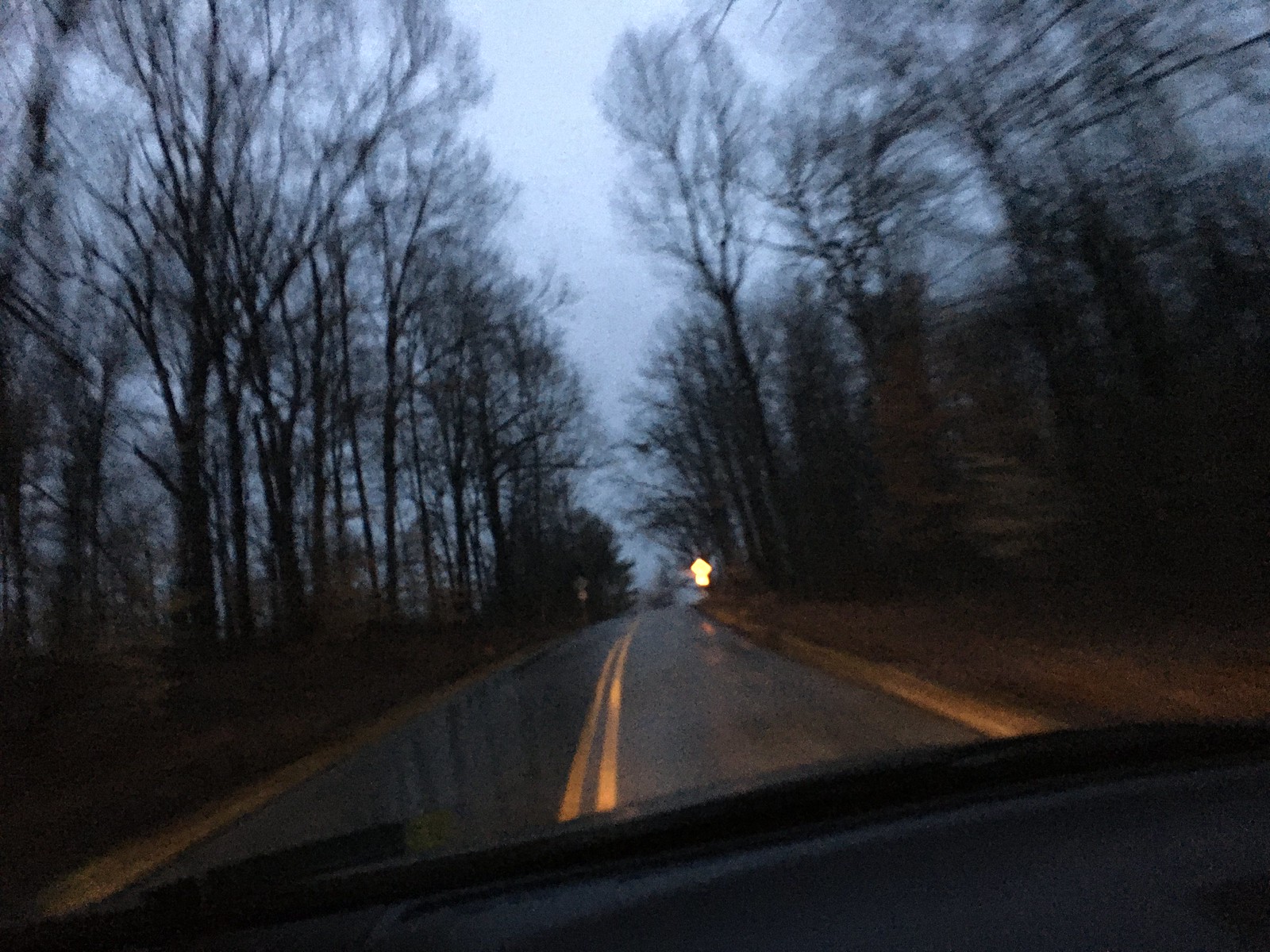This slightly rectangular, horizontally framed image captures a nighttime scene through the windshield of a vehicle. The shot is slightly angled, adding a hint of dynamic tension to the composition. The foreground, where the vehicle’s headlights illuminate the road, is sharply in focus. The two-lane road, marked by a double yellow line, stretches into the distance. In the center of the frame but farther away, the headlights reveal a yellow square traffic sign. On either side of the road, tall and barren trees create a haunting silhouette, appearing to lean slightly to the left due to the angle of the shot. The overall image is quite blurry, except for the clear, well-defined stretch of road immediately in front of the vehicle, emphasizing the isolation and depth of the night journey.